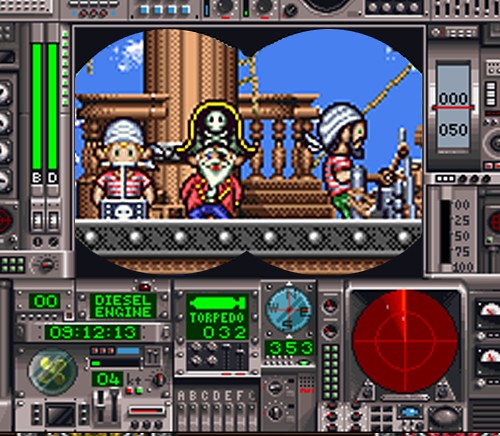This image is a detailed screenshot from the Japanese-exclusive Super Nintendo game, Bing Bing Bingo. The scene captures a vivid 8-bit visual of a pirate-themed scenario where the player is looking through a telescope, focusing on a pirate crew aboard a wooden ship. In the scope's circular view, three pirates are displayed prominently, each adorned in traditional pirate attire: one wears a red coat, blue pants, a long white beard, and a typical pirate hat with a skull and crossbones, while the other two crew members don red and white striped shirts and white headbands. The scene includes detailed elements such as a massive wooden mast, surrounding wooden beams, and spokes.

In the foreground, the game's HUD (Heads-Up Display) is intricate and functional, showcasing a diesel engine readout, torpedo inventory, and various other metrics displayed in fluorescent green. The interface is packed with silver-colored gadgets, including levers labeled A through G, numerous buttons, a fan, a compass, and a bright red map highlighting different locations. The mix of pirate imagery and mechanical controls creates an immersive, complex gameplay environment reflective of the vintage 8-bit gaming era.